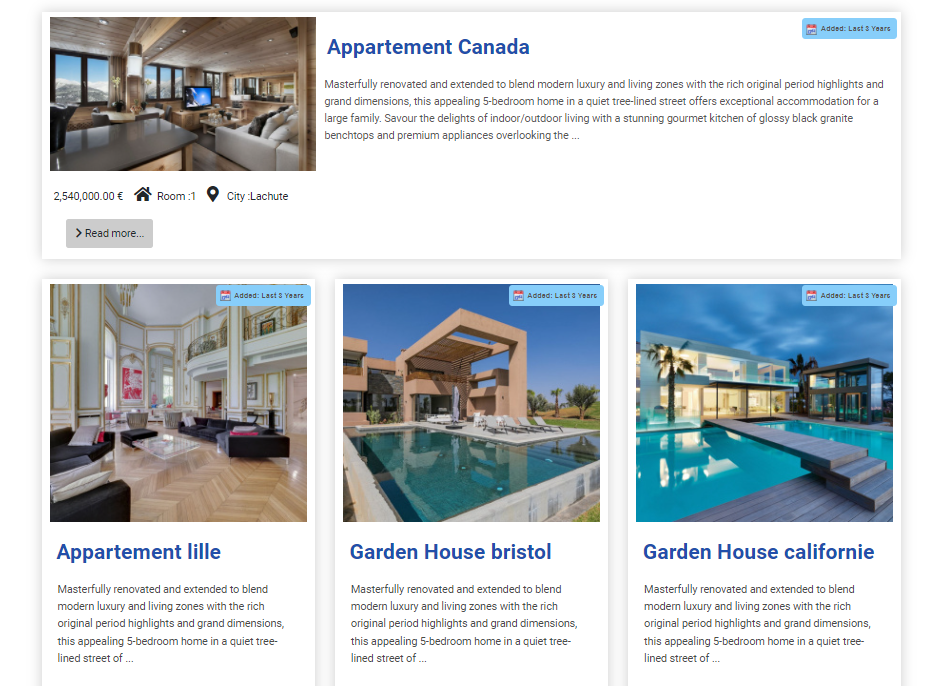The top left corner of the image showcases a photograph labeled "Apartment Canada." This residence has been masterfully renovated and extended to seamlessly blend modern luxury with its original period features, creating a harmonious living environment. This exquisite five-bedroom home, situated on a tranquil, tree-lined street, offers substantial accommodation perfect for a large family. The residence features an indoor-outdoor living area highlighted by a stunning gourmet kitchen with glossy black granite countertops and top-of-the-line appliances.

Below the primary photograph, there's an image of a spacious living room bathed in natural light, featuring numerous windows, comfortable couches, and a large flat-screen TV. The price listed for the house is €2,540,000, under the label "house," with one room specified. This property is located in Lachute.

Further below, there are three photographs arranged in a row. The first is labeled "Appartement," located in Lille. It too has been masterfully renovated to combine modern luxury with historical architectural elements, providing an appealing five-bedroom home on a peaceful tree-lined street. The next photo is labeled "Garden House, Bristol."